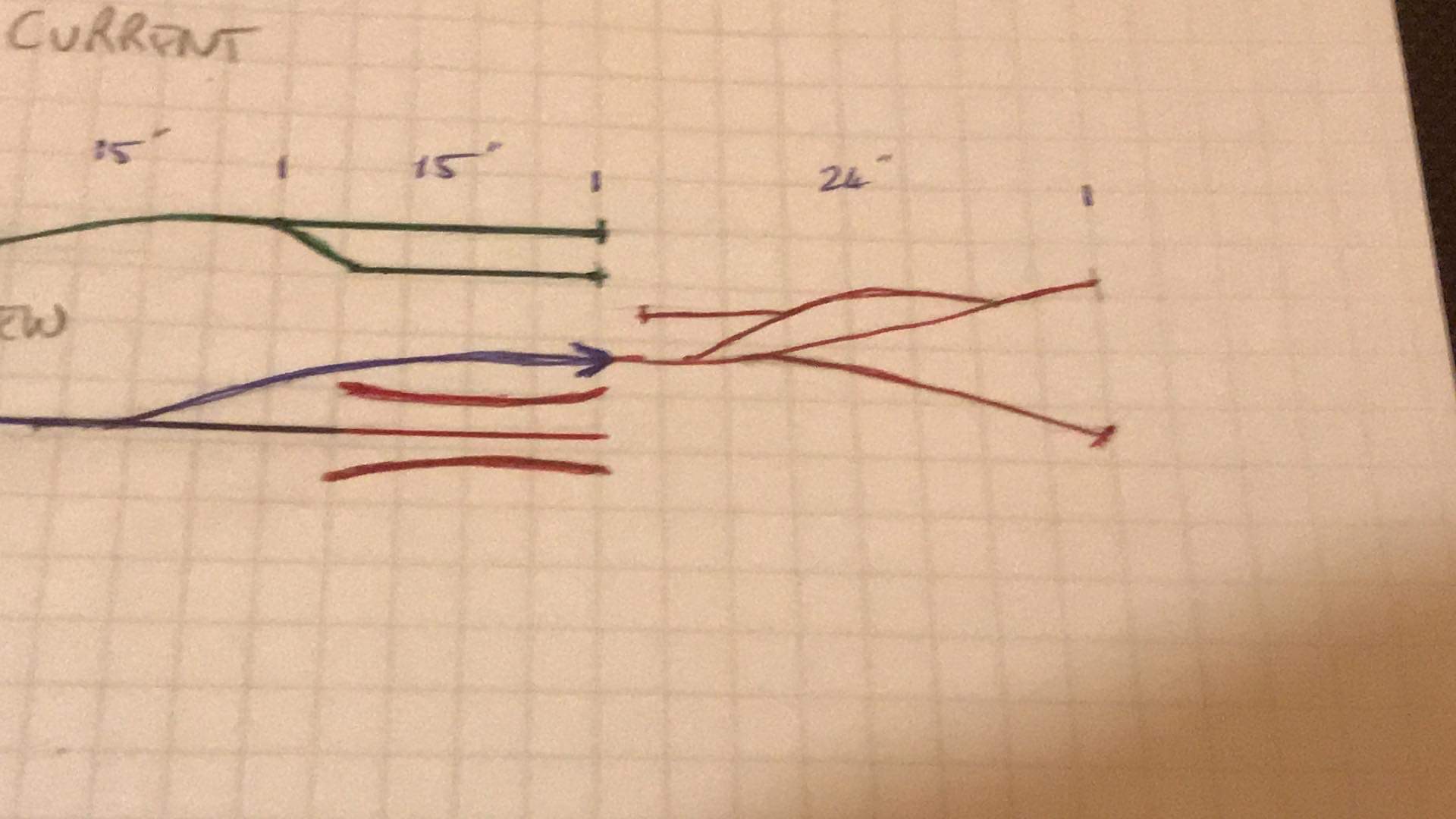The image is a detailed close-up of a piece of squared paper, typical of those found in mathematics or electronics textbooks, indicative of an academic setting. The grid pattern covers the entire page, providing a structured background for the notes. At the top of the page, the word "Current" is handwritten, suggesting the focus of the notes.

Below this title, various circuit diagrams are meticulously drawn using different colored pens—green, blue, and red. These diagrams feature lines that intersect and diverge, illustrating the complex layout of the circuits. Each line is annotated with measurements, though there is an ambiguity between whether these denote feet or inches; specifically, measurements like "15 feet," "15 feet," and "24 feet" are written, which could alternatively be "15 inches," "15 inches," and "24 inches."

The diagrams are detailed with precise annotations that likely explain the flow and dimensions of the circuit components. A shadow is cast on the bottom right of the page, suggesting the image is illuminated from behind and to the left of the camera's viewpoint, adding depth to the scene.

Overall, the image captures a snapshot of an electronics student's detailed and colorful study notes, replete with technical diagrams and essential annotations.